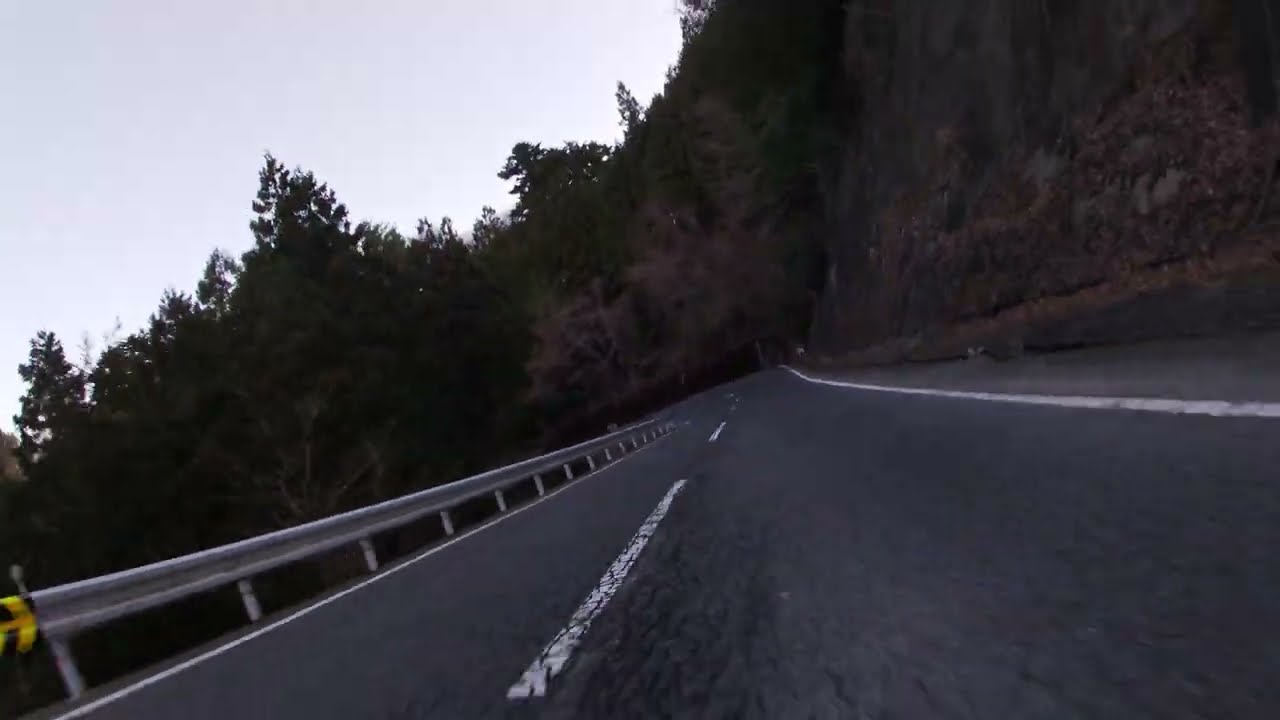This landscape photograph captures a curving, two-lane highway nestled in mountainous terrain. The road, composed of asphalt, features solid white lines on the edges and dashed white lines down the center. A silver guardrail runs along the left side, providing a safety buffer against the steep terrain. To the right, a rugged hillside rises, dotted with tall trees, possibly pines, growing amidst the rocky outcrops where the road was carved out. The scene is cloaked in shadows cast by the mountain, creating a darker ambiance despite it being daytime. There is a noticeable patch of blue sky in the upper left corner, partially obscured by clouds and mountains, with the sun hidden and casting a dim light over the scene. A small splash of yellow appears at the bottom left, likely a road sign indicating a sharp curve ahead. The photo's angle is slightly tilted, adding a dynamic feel to the composition.